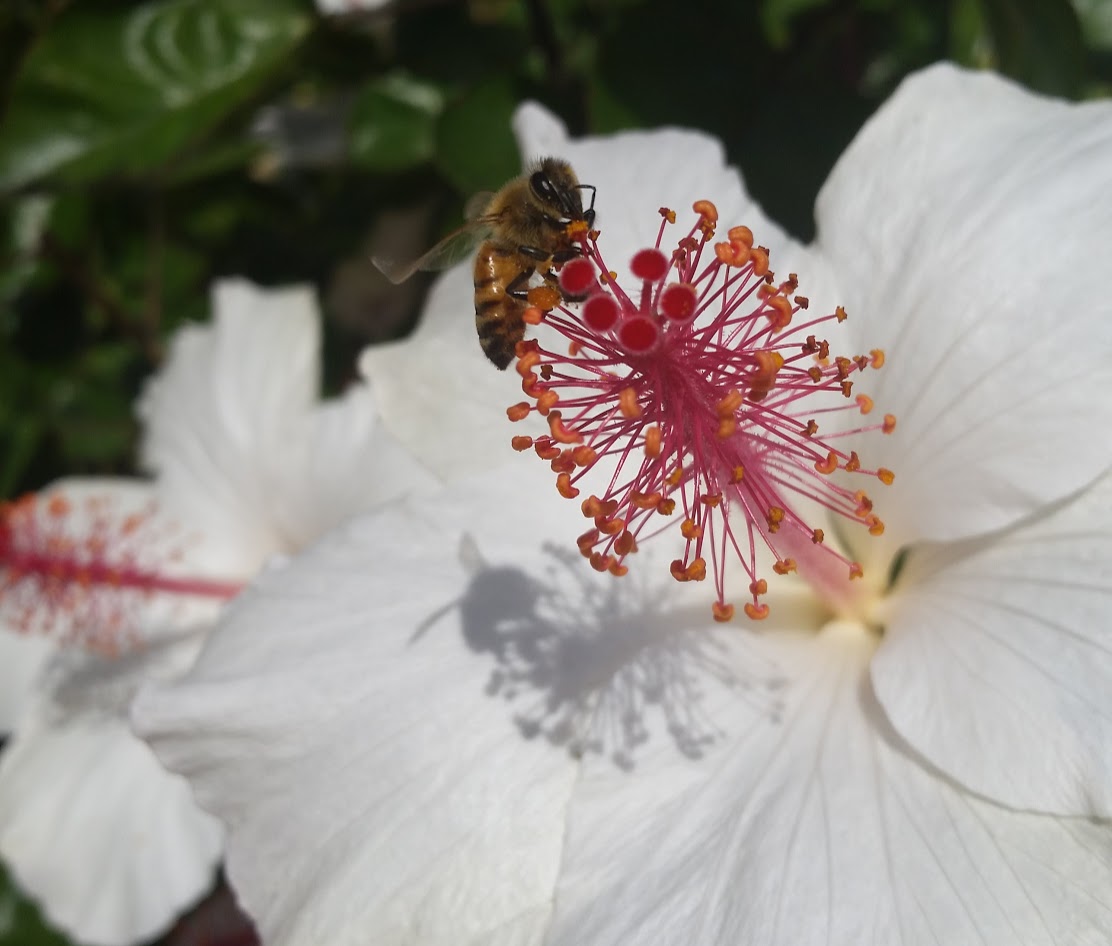In this high-quality, color photograph, a vividly detailed close-up captures the intimate beauty of a white flower in full bloom, set against a backdrop of darker green, shiny leaves. Dominating the foreground are two white flowers; the larger of the two is accentuated by a bee busily collecting pollen. This larger flower features intricate veining on its green leaves, and its prominent center protrudes outward, showcasing a captivating mix of red, orange, and pale yellow hues. The bee, with its fuzzy, light brown upper body, darker shiny brown lower part, and clear, thin wings, is framed against the striking red and orange stamen, which culminate in circular tips. The bee's shadow and the vivid center of the flower reflect off the white petals, adding a dimensional quality to the image. Pollen is visibly scattered across the flower's center, emphasizing the natural symbiosis between the bee and the bloom. Another flower and more green foliage gently blur into the background, enhancing the depth and focus of this nature-rich scene.